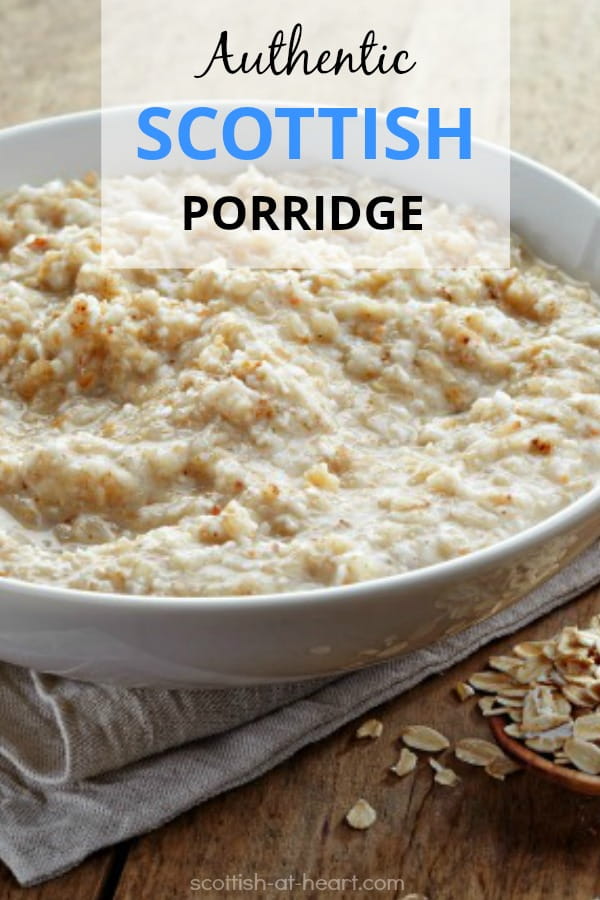In this image, a freshly made bowl of traditional Scottish porridge is prominently placed at the center. The white bowl contains a light beige, soft-textured oatmeal, showcasing its freshly-cooked, hearty consistency. The finely detailed photograph highlights the coarse, chunky texture of the porridge, emphasizing its wholesome appeal. Above the bowl, a transparent white text box announces "Authentic Scottish Porridge," with the word "Authentic" displayed in black script lettering, "Scottish" in bold blue uppercase, and "Porridge" also in bold black uppercase. The setting includes a brown wooden table adorned with a grey linen napkin, and a scattering of oats can be seen at the corner, adding a rustic touch. At the bottom of the image, "scottishatheart.com" is subtly printed in tiny white letters. The overall scene is bright, clear, and inviting, fully focusing on the comforting simplicity of this traditional Scottish dish.